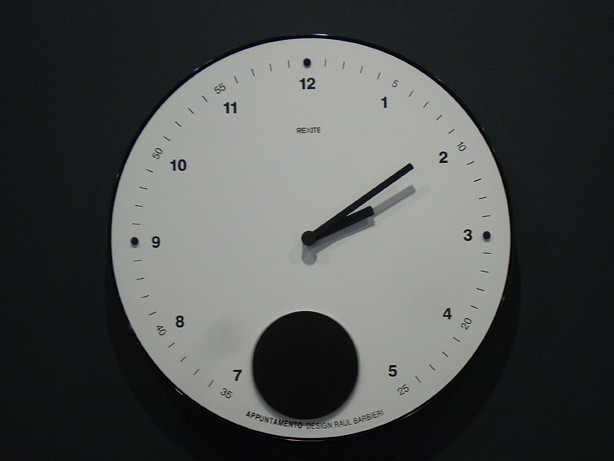The image showcases a minimalist and modern analog clock mounted on a nearly black wall. The clock features a white face with a thin black border that reflects light, emphasizing its sleek design. The clock face is adorned with simple black lines representing the hours from 1 to 12, with longer lines indicating the hours and shorter ones for minute markers. These minute markers are further divided into 5-minute increments, with additional numerical indicators for 5, 10, 15, 20, 25, and so on, up to 60.

At the center of the clock is a prominent black circle, likely serving both as a design element and to conceal the movement mechanism. The clock hands are black, sleek, and contemporary, showcasing a streamlined design. The time shown is approximately 10 past 2, with a subtle grey shadow cast by the clock hands due to overhead lighting.

Text appears just beneath the central black circle, indicating the design and designer of the clock: "A Pimento Design Raoul Biberi," elegantly printed in black. This text adds a touch of sophistication and authenticity to the piece.